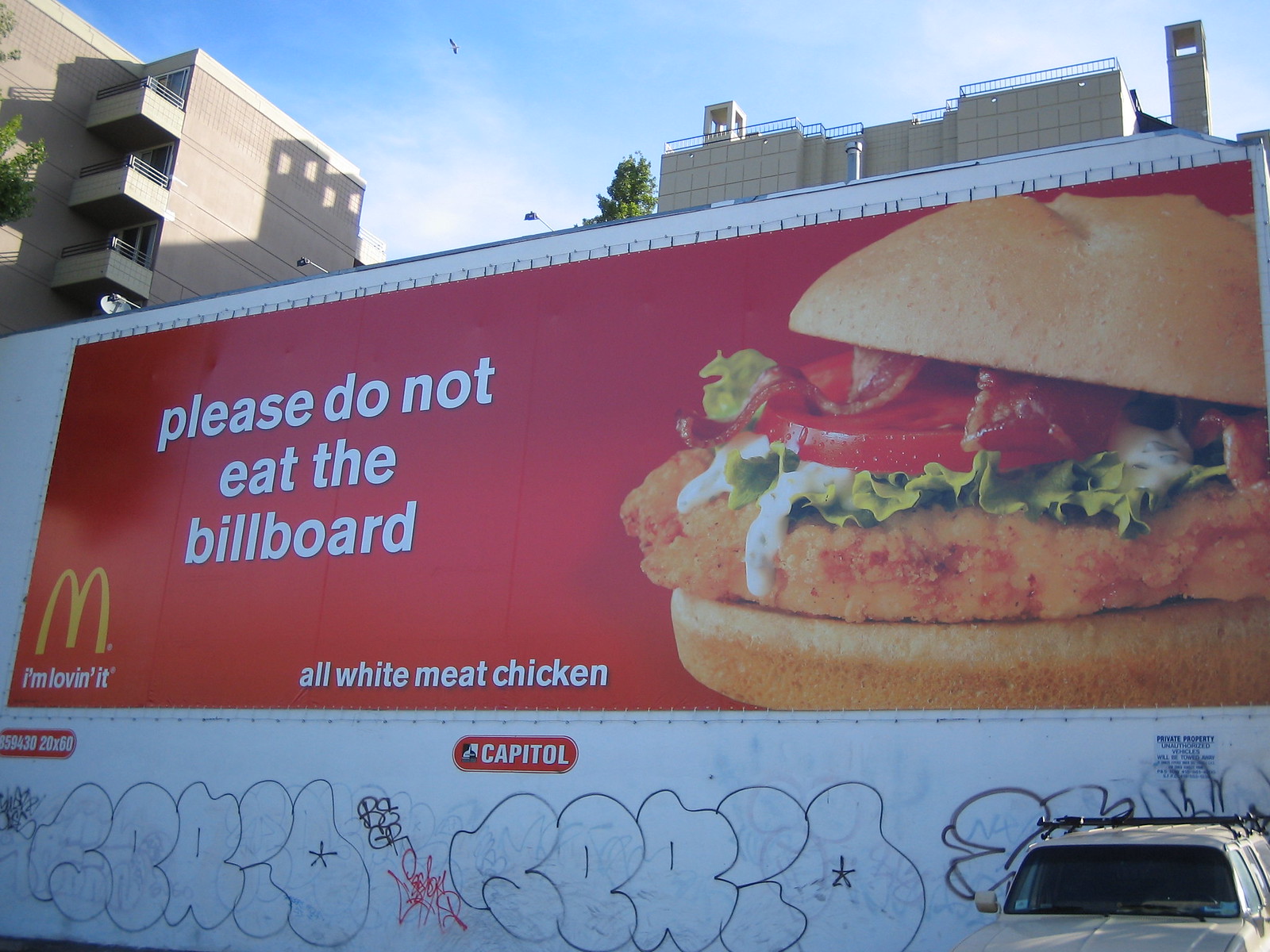This outdoor city scene features a prominent McDonald's billboard occupying the foreground of a rectangular landscape image. The billboard, slightly angled with the upper right higher than the lower left, commands attention with its vivid red background and bold white text. It reads, "Please do not eat the billboard," with "all white meat chicken" directly below. To the right, an enlarged, mouth-watering image of a McDonald's chicken sandwich is displayed, complete with a pulled-back bun, crispy chicken patty, fresh lettuce, ripe tomato, mayonnaise, and bacon. A small, red cylindrical logo with the word "Capital" marks the bottom of the billboard, likely indicating the owner.

Below the billboard, a white wall with illegible, bubbly-lettered graffiti and the odd red scribble adds an urban touch. The lower right corner reveals the top part of a white truck backed into a parking space. In the background, a deep blue sky frames several buildings. One light stone-colored building on the left features three visible balconies, suggesting residential use. Adjacent to it is a taller, brighter building on the right. Additionally, a smaller white building below sports the iconic red McDonald's sign, reinforcing the brand's presence. Together, these elements create a layered and vibrant urban landscape.